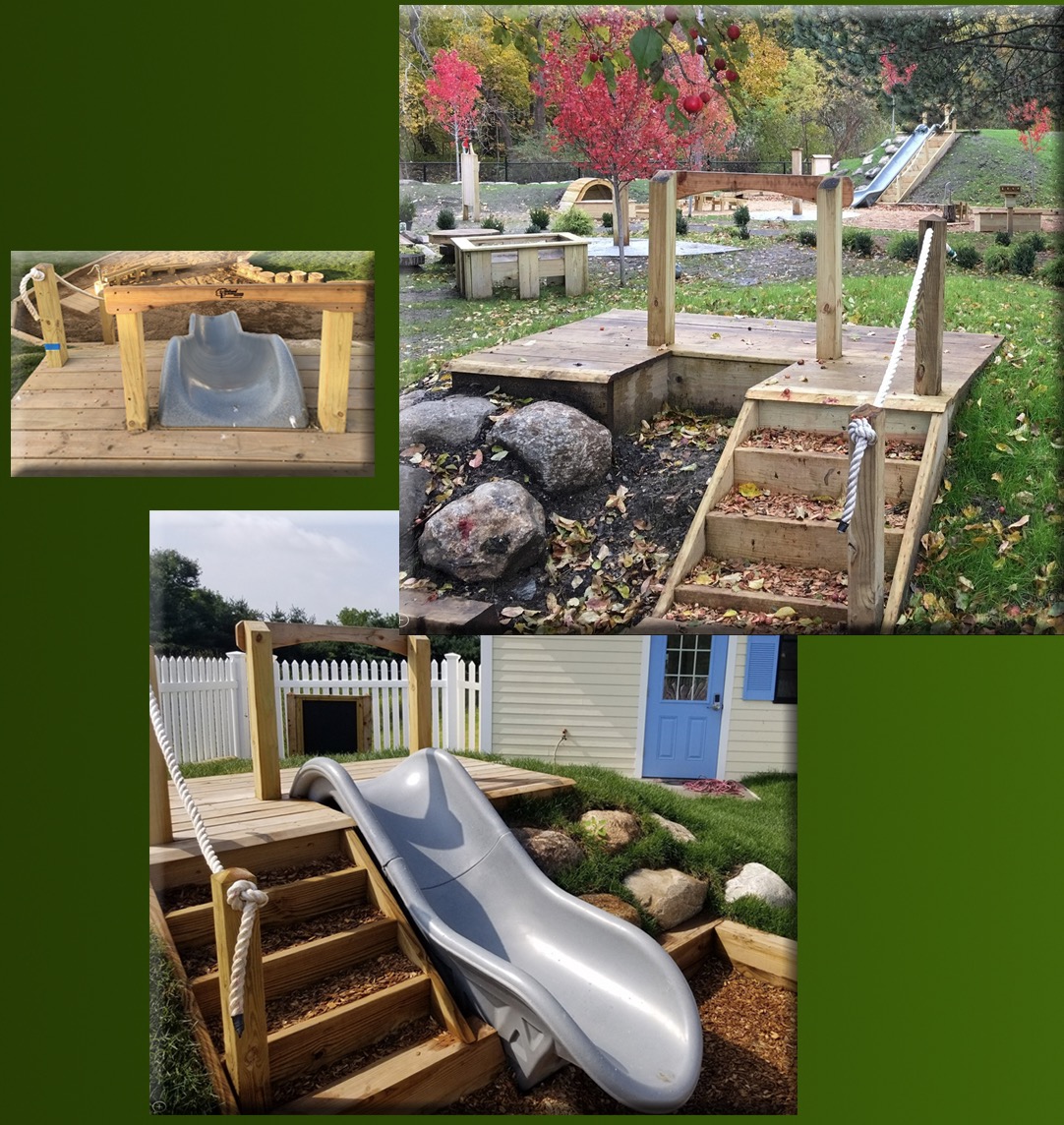The image is a detailed montage of three photographs set against a green background. The largest photograph, located in the upper right, captures a playground or backyard scene featuring a wooden playset with steps leading up to a small wooden platform. In front of the steps are large rocks, and surrounding the structure is a lush green lawn. Additional wooden elements, including a planter and a bridge-like structure, are seen, and the far right showcases stairs amidst more grassy areas. The backdrop reveals a vibrant autumn landscape with red, yellow, and green leaves on the trees.

In the bottom left of the montage, there is a close-up angle of a small plastic slide with wooden steps leading up to the platform, emphasizing a detailed view of the playset. A blue shed appears partially visible behind the slide, hinting at a residential backyard.

The upper left photograph offers a top-down perspective of the same slide area, showing the platform's view from above. Fallen leaves are scattered on the steps, accentuating the autumn setting. Across all images, cohesive elements such as the green grass, wooden structures, and surrounding decorations are illustrated in great detail, showing the slide in various stages either of assembly or use.